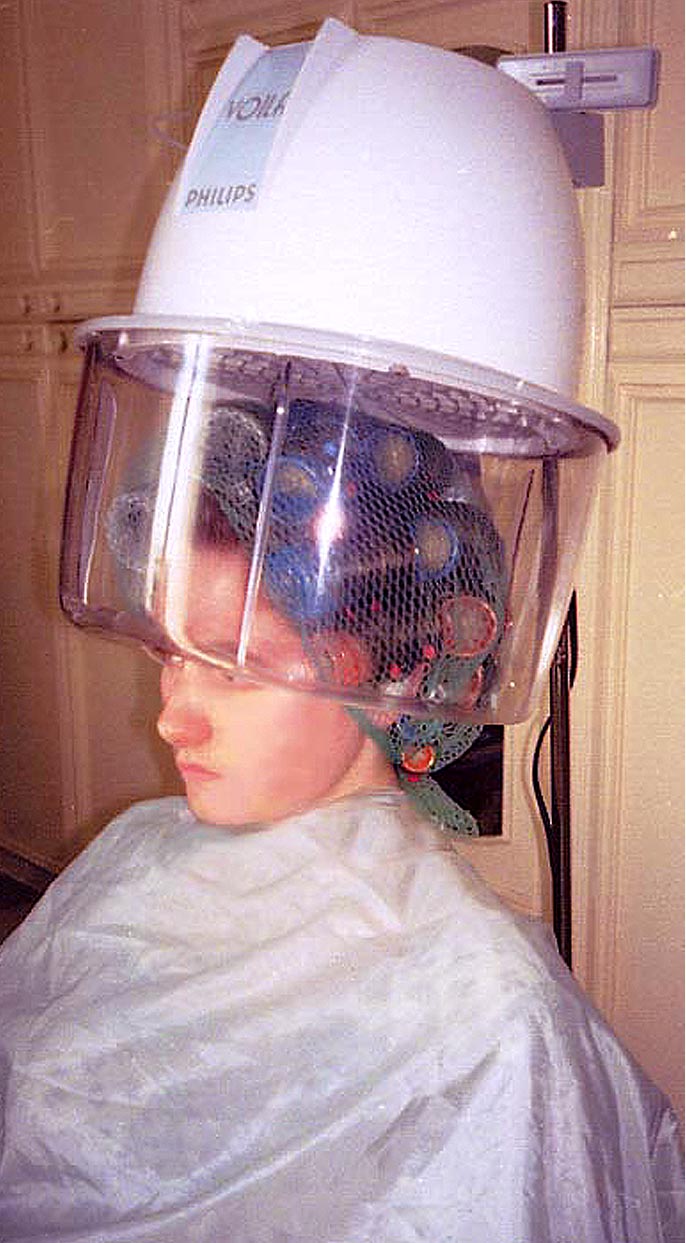The vintage photograph captures a woman at a hair salon, seated under an old-fashioned hair perming machine. The device, labeled "Voila Phillips" on the white plastic dome, features a clear circular shield that covers the woman's head and hair. Her hair is held in blue, red, and possibly pink and orange curlers, secured with red sticks and covered by a mesh hairnet. The woman, with a light skin complexion and dark hair, wears a grayish-white plastic cape to protect her clothes. She appears to be looking slightly to the left, her face showing a stern expression. The background is a white wall filled with cabinets and door handles, adding to the vintage ambiance of the scene.